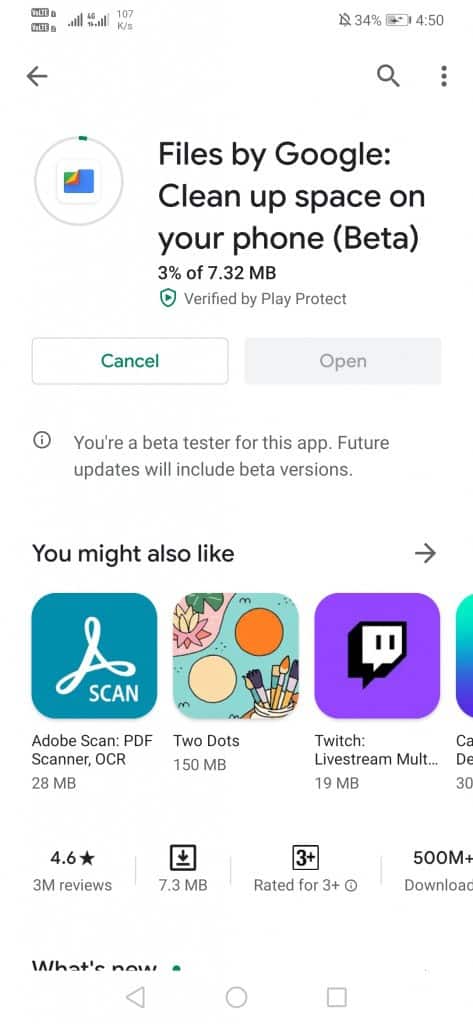In this detailed depiction of a phone screen, an individual is seen downloading a beta version of the "Files by Google" app, designed to clean up space on the device. The screen's upper section displays standard status icons: a left-pointing arrow, the text "LETE" potentially indicating a UI glitch, a clock showing 4:50, a muted sound icon, 34% battery life with a charging indicator, 4G connectivity, and a data transfer rate of 107K/s.

Beneath this, a search icon and a three-dot menu are visible. The app being downloaded, "Files by Google - Clean up space (Beta)," is shown along with its progress - 3% of 7.32 MB downloaded. This app is verified by Play Protect. There are two buttons below: a green "Cancel" button and a greyed-out "Open" button, which remains inactive due to the minimal progress indicated by the download's progress bar.

A message confirms the user is a beta tester for this app, hinting at receiving feature updates in the beta phase. Suggestions for alternative or additional apps include Adobe Scan, Two Dots, and Twitch, with an arrow allowing exploration of more options. Adjacent details provide the app’s rating of 4.6 stars based on three million reviews, its size of 7.3 MB, a minimum age rating of 3+, and over 500 million downloads. The bottom of the screen partially reveals a "What's new" section.